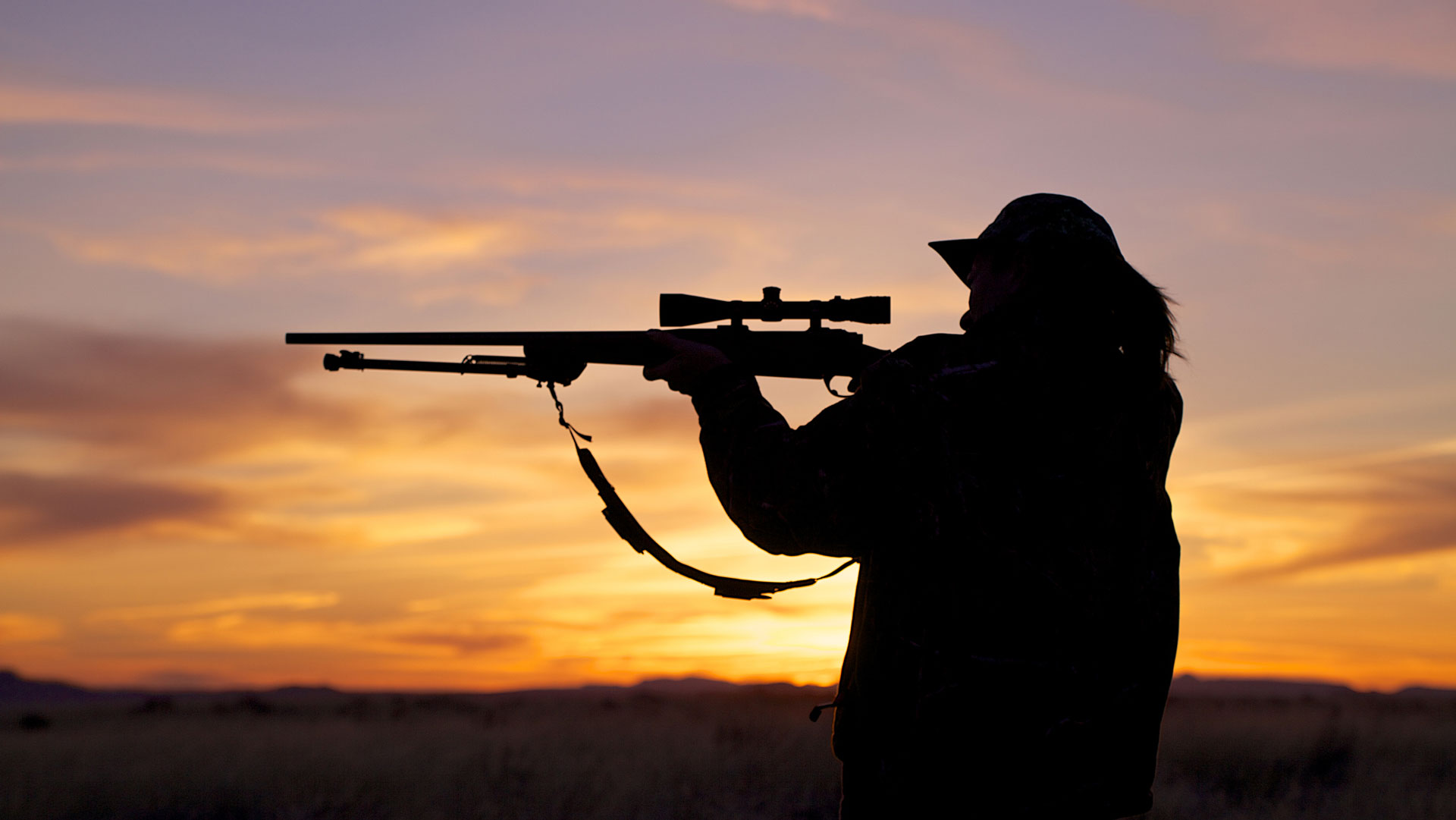The photograph captures the dramatic silhouette of a person aiming a scoped rifle against a vivid sunset sky. The silhouetted figure, possibly a man, appears to be wearing a hat and pointing a bolt-action rifle equipped with a tripod and sling towards the left side of the image. The person is in a side view, making it difficult to discern specific facial features but allowing the observer to see the outline of their head, arms, and rifle. The backdrop features a stunning gradient sky starting with bright yellow and orange hues near the setting sun, transitioning to darker reds and eventually a bluish tint higher up. Scattered white clouds reflect the sunset's colors, and a faint mountain silhouette is visible in the distant background. The person's finger seems to be on the trigger, suggesting they are ready to fire. This carefully composed shot highlights the serene yet intense moment against the natural beauty of dusk.